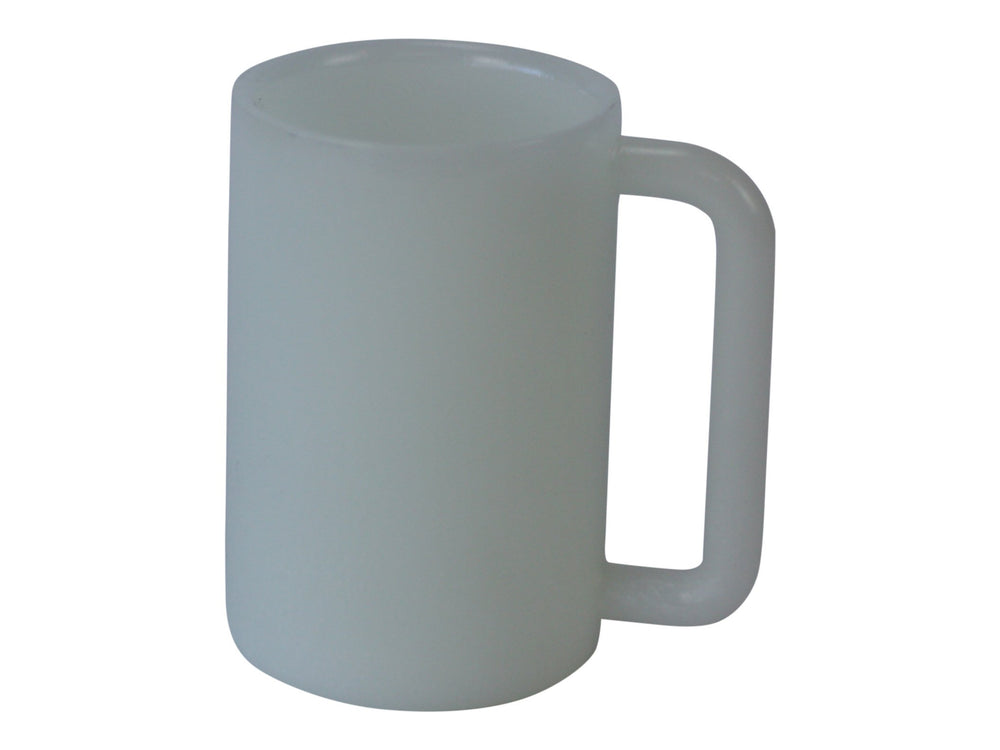The image showcases a tall, light gray mug, likely made of glass, ceramic, or possibly borosilic tempered glass, with a contemporary style. The mug has a cylindrical shape and a smooth, unadorned surface that reflects light slightly on the back rim, giving it a pristine and polished appearance. The handle is large, making a D shape that extends almost from the top to the bottom of the mug, and it is slightly chamfered at the edges. The handle's substantial size adds to the mug's unique and somewhat abnormal aesthetic. The entire scene is set against a white background, emphasizing the mug’s minimalist design and subtle shading. The image appears almost like a 3D render or a piece of modern art, focusing solely on the mug with no other elements to distract from its form and function.